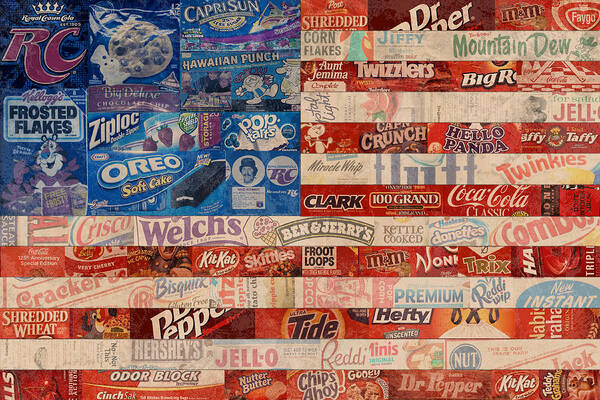The image is a detailed collage that intricately forms the image of an American flag using various brand logos and product wrappers. The flag’s red and white stripes are made up of an array of recognizable brands. The red stripes feature brands like Dr. Pepper, M&M’s, Twizzlers, Coca-Cola, 100 Grand bars, Big Red, Captain Crunch, and Twinkies, while the white stripes display brands including Mountain Dew, Jell-O, Ben & Jerry’s, Welch’s, and Twinkies. The top left corner, where the stars of the American flag would typically be, is a blue rectangle filled with more brands such as Oreo, Frosted Flakes, Ziploc, Capri Sun, and Hawaiian Punch. Each color section of the flag is crafted by merging these colorful logos and brand names, creating a visually striking and patriotic pastiche.